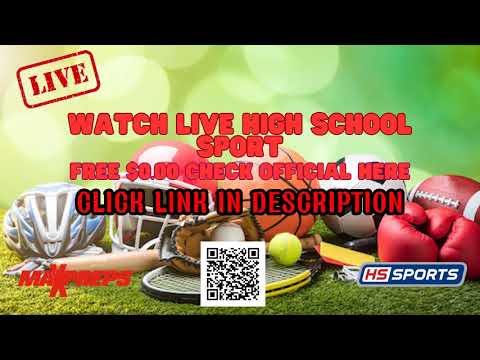The image appears to be an infographic or TV advertisement promoting high school sports. Displayed on a backdrop of lush green turf, various sports equipment such as a bike helmet, football helmet, basketball, baseball glove, soccer ball, tennis ball, tennis racket, boxing glove, and football are spread out. The upper portion of the image is blurred, showcasing various shades of green with circular disks resembling out-of-focus light sources. The image is framed by two black horizontal bars, giving it a wider appearance. 

In the upper left corner, a red stamp reads "LIVE," indicating real-time broadcast. Below it, red text reads: "Watch Live High School Sport for Free - $0.00. Check official here. Click link in description." A QR code is positioned near the bottom center of the image, flanked by additional text. To the right of the QR code, it says "HS Sports" with "HS" in red and "Sports" in white. On the left, there's indistinct red text, potentially starting with "M" or "Max." The overall layout and vibrant colors effectively capture the dynamic nature of high school sports events.